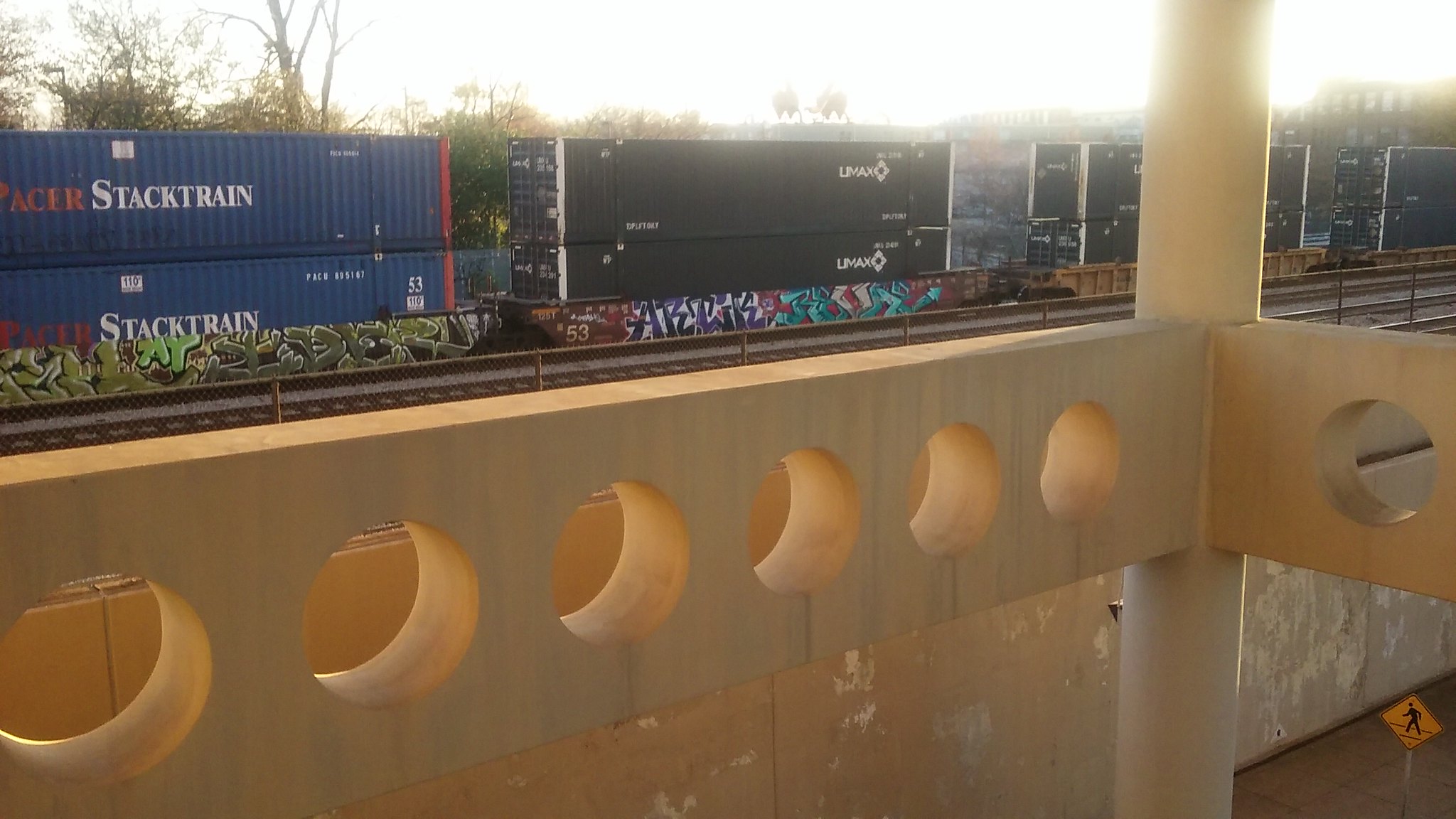This photograph captures a side view from a balcony overlooking a train track, where stacked boxcars traverse a slightly diagonal route. Against a bright, white sky punctuated by a row of trees, a series of train cars dominate the composition. On the left, two blue cars emblazoned with "Pacer Stack Train" contrast sharply against their darker counterparts. To their right, two black boxcars labeled "LMAX" are followed by additional black boxcars, creating a seamless line of cargo. Each boxcar stack consists of two cars, catching a glimpse of graffiti that adorns the sides. 

In the foreground, a prominent rectangular railing with circular cutouts in the middle frames the view, leading the eyes towards the train. A yellowish concrete block emerges from the bottom left corner, featuring six cut-out circles, and is intersected by a substantial concrete pillar that almost reaches the top of the image. Adjacent to this pillar, another segment of the concrete block extends rightward, with a single circular cutout. Finally, a yellow pedestrian walk sign is visible in the bottom left, hinting at the urban setting below the balcony.